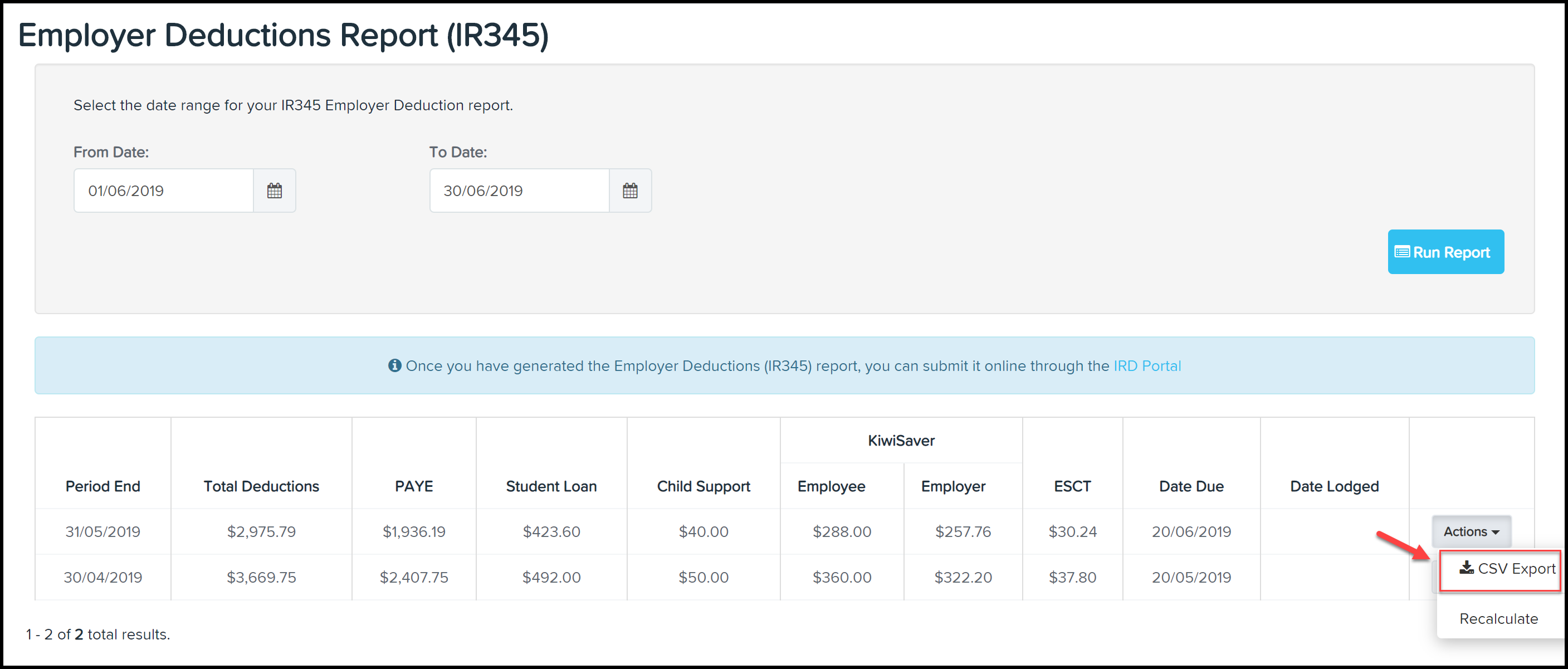The image in question is an online interface for generating an "Employer Deductions Report," identified by the code "IR 345." The layout begins with a black outlined box at the very top of the interface, where "Employer Deductions Report (IR 345)" is prominently displayed in the top left-hand corner.

Directly below this title, there are instructions in small black letters that read: "Select the date range for your IR 345 employer deduction report." Subsequently, there are two input fields labeled "From" and "To" for date range selection. The "From" date box is populated with "01/06/2019" and the "To" date box is filled with "30/06/2019."

At the bottom right-hand corner of this date selection box, there is a blue button labeled "Run Report." Clicking this button will generate the report based on the specified date range.

Further down the interface, a light blue banner spans across the width of the screen. The banner instructs users: "Once you have generated the Employer Deductions IR 345 report, you can submit it online through the IRD portal."

Below this banner, the interface provides detailed information fields related to the report. These fields include:
- Period End Dates
- Total Deductions
- Pay
- Student Loan Amount
- Child Support Amount
- Employee Contributions
- Employer Contributions
- Employer Superannuation Contribution Tax (ESCT)

Each of these fields is intended to be filled with relevant data summing up the employer's deductions for the given period.